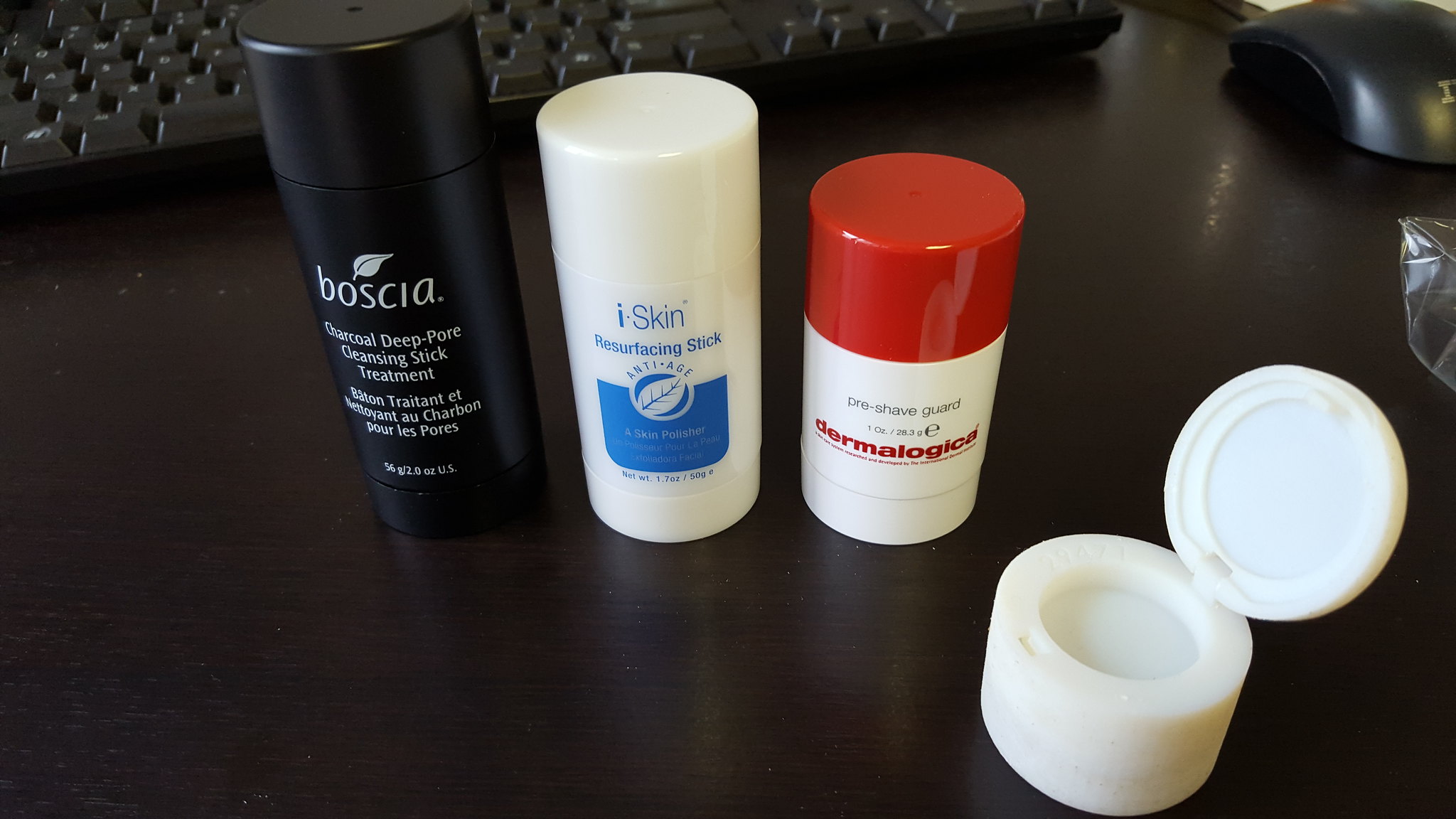In this image, a dark brown tabletop serves as the background for an arrangement of various items. At the top left corner, a keyboard stretches almost entirely across the top of the scene, accompanied by a black mouse positioned directly to its right. 

In the foreground, a series of cylindrical containers can be seen. The first one is a bottle of Boscia Charcoal Deep-Pore Cleansing Stick Treatment, identified by its green leaf logo. The text on the bottle includes the product name in both English and another language.

Adjacent to the Boscia bottle is another cylindrical container labeled iSkin Resurfacing Stick. This container features a reversed leaf design inside a blue circle, alongside a blue banner with rounded corners displaying additional product details.

Next in line is a cylindrical container with a red cap and the brand name Dermalogica in red letters. Black text is also visible on the upper portion of this white bottle, which is identified as a pre-shave treatment.

Lastly, to the right of the Dermalogica bottle, there is a shorter cylindrical container with a flip-top lid that is currently open. The interior appears white, though it is unclear whether this color is from the container itself or its contents.

These descriptions provide a detailed overview of the objects placed on the tabletop, highlighting their arrangement and distinctive features.